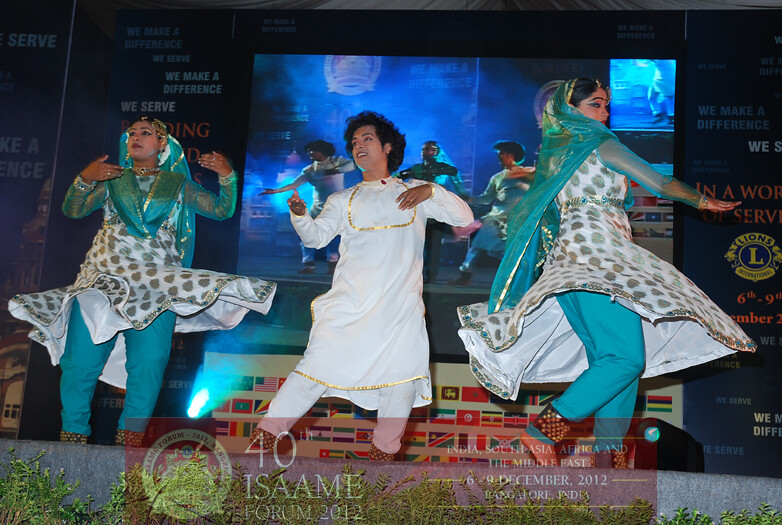The image depicts a vibrant scene of three people—two women and a man—performing a dance on a stage, likely during an Islamic music ceremony. The women, positioned on either side, are wearing long dresses adorned with blue and green dots, complemented by turquoise pants underneath and a sheer blue shawl draped over their heads and down their backs. They have thick anklets around their ankles. The man, standing between them, is dressed in a flowing white tunic trimmed with gold, paired with white pants. Behind them is a large TV monitor reflecting their live performance and flanked by a wall adorned with numerous international flags, indicating a diverse and inclusive event. At the bottom of the image, the text reads "40th ISAME Forum 2012, India, South Asia, Africa, and the Middle East, 6 through 9 December 2012, Bangalore, India," marking the occasion of the 40th ISAME Forum. The scene vibrantly captures the cultural richness and celebratory atmosphere of the event.